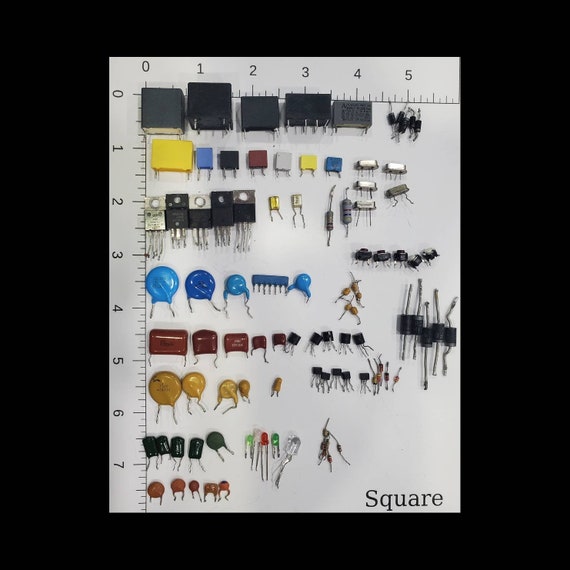This detailed photograph showcases a collection of various electronic components meticulously arranged on a white grid background, which measures 6 inches by 8 inches. The grid features ruler markings along the left and top edges, with the left side marked from 0 to 7 inches and an additional inch extending beyond, though not numbered, indicating an 8-inch height; similarly, the top edge is marked from 0 to 5 inches, extending to an unnumbered 6-inch width. In the bottom right corner of the grid, the word "square" is printed in bold black text.

The components, possibly for a motherboard or intricate circuitry, are laid out with precision. At the top, along the 6-inch axis, are square-shaped transistors of various sizes, starting at the 0-inch mark and stretching to the 4-inch mark, some featuring visible silver pins. Moving down, there are clustered smaller transistors around the 5-inch mark. Scattered across the grid, these components come in a variety of shapes and colors: yellow, blue, brown, black, gray, silver, burgundy, and red. Rectangular transistors with rounded edges stand out in burgundy and red, while circular transistors, which resemble insulated wires, appear in shades of cyan, dark blue, mid-blue, dark and light brown, and yellow.

The layout follows a systematic arrangement, with larger components at the higher rows, decreasing in size as you move downward. At the bottom, a grouping of transistors resembles colorful Christmas bulbs, adding a unique visual element to the composition. This assortment of carefully organized electronic parts not only highlights the diversity in size and shape but also the colorful array of components found in modern circuitry.